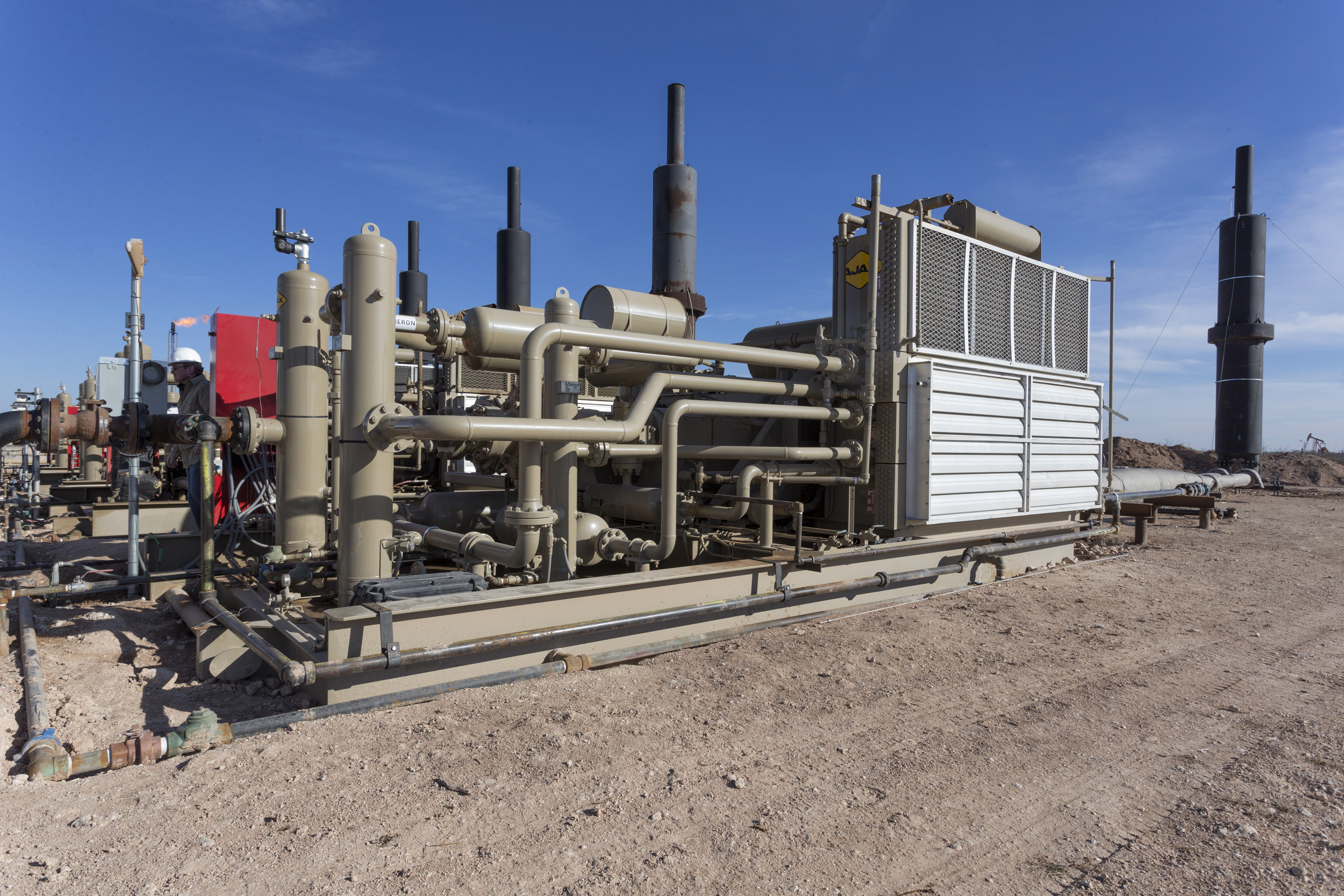This photo depicts an outdoor scene on a sunny day with a clear blue sky and minimal cloud coverage, set in a barren, desert-like landscape with rocky, sandy soil. The central focus is on an extensive piece of industrial machinery, possibly part of a mining or natural gas facility. The machinery includes numerous interconnected pipes and hoses, predominantly painted in a beige or light gray color. Prominent within the setup is a large steel radiator or air handling unit, which features four silver, vent-like sections resembling air conditioner filters and additional white, slatted segments. A black tank with two white stripes and string extending to the ground is also visible. Nearby, a red machine and various pipelines add complexity to the apparatus. Off in the distance, background details include dirt hills and a tall tower with a flame at its apex, indicating potential natural gas operations. The scene captures a functional, industrial setup against a stark, expansive landscape.